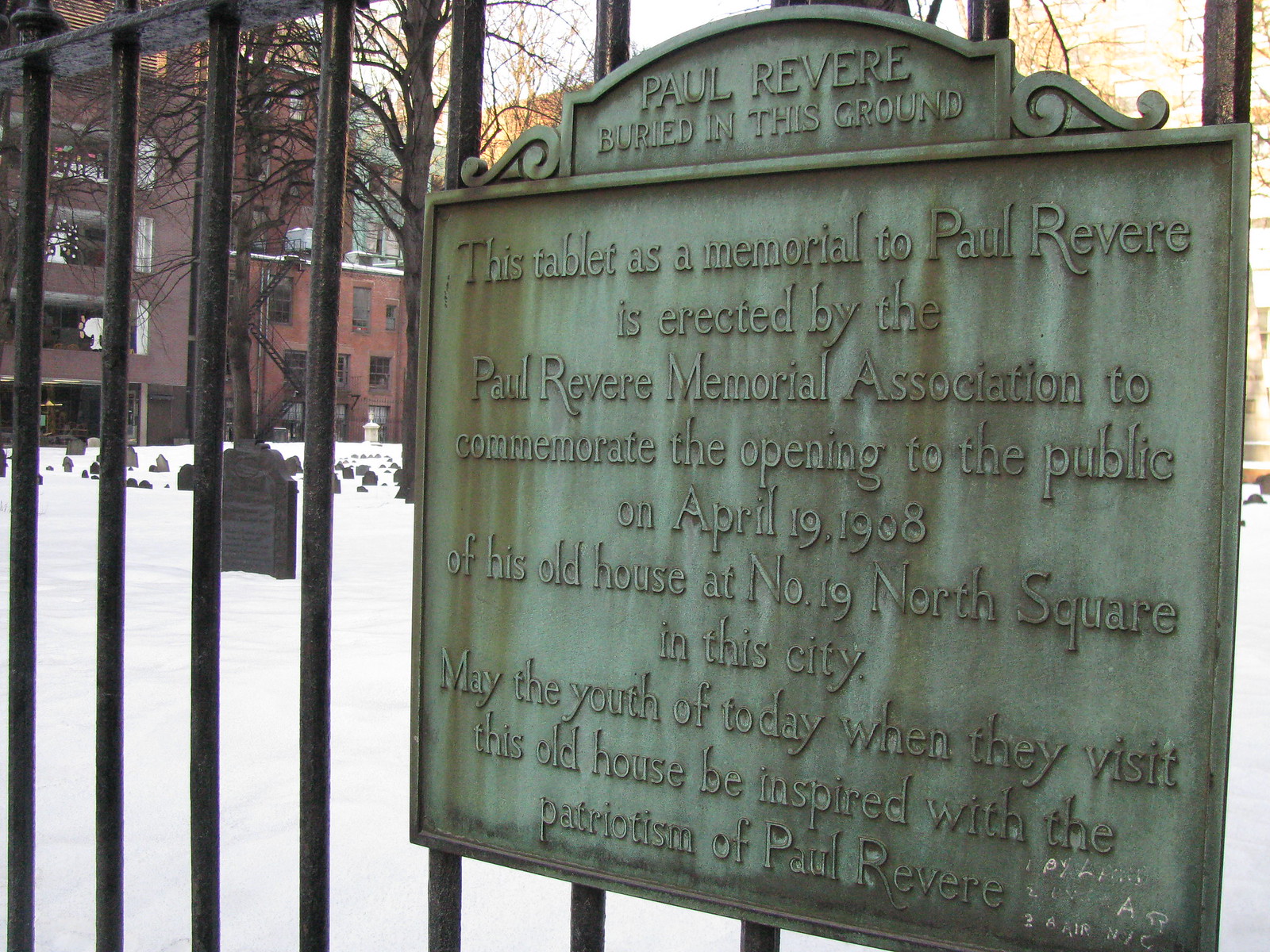This photograph captures a close-up view of a weathered metal plaque mounted on an iron fence outside a snow-covered cemetery. The top of the plaque reads: "Paul Revere buried in this ground." The inscription continues, stating that the plaque was erected by the Paul Revere Memorial Association to commemorate the public opening of Paul Revere's old house at 19 North Square, Boston, on April 19, 1908. It also includes a message hoping that visiting youth will be inspired by Revere's patriotism. The plaque spans from slightly left of center to the right edge of the frame. To the left, several gravestones are visible against a snowy background. Beyond the cemetery, there are tall, red brick buildings, suggesting the urban setting of downtown Boston.